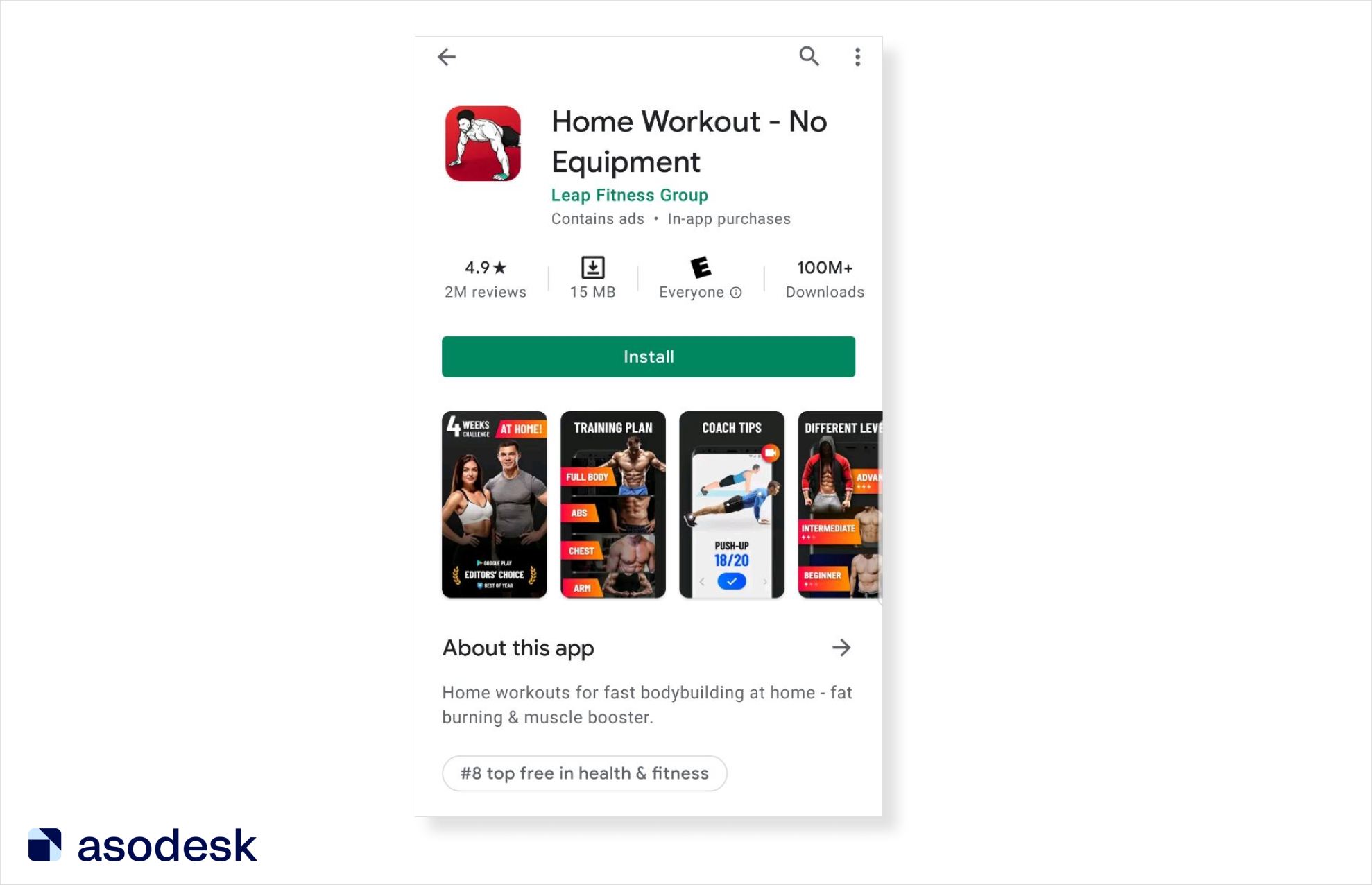The image is a screenshot of the Apple App Store featuring the 'Home Workout - No Equipment' app. In the upper left corner, there is a left arrow icon, while the upper right corner shows a magnifying glass (search icon) and a three-vertical-dots (more options) icon. Below these icons, a thumbnail image displays a man performing push-ups, representing the app. The app is named 'Home Workout - No Equipment,' developed by Elite Fitness Group. It includes mentions of ads and in-app purchases. The app boasts an impressive rating of 4.9 stars based on 2 million reviews, has a size of approximately 15 MB, is rated E for everyone, and has been downloaded over 100 million times. A prominent green 'Install' button is visible. Further down, there are several screenshots showcasing different pages of the app, followed by a section titled 'About This App.' Additionally, the app is ranked eighth in the top free apps within the Health and Fitness category on the ASO desk.